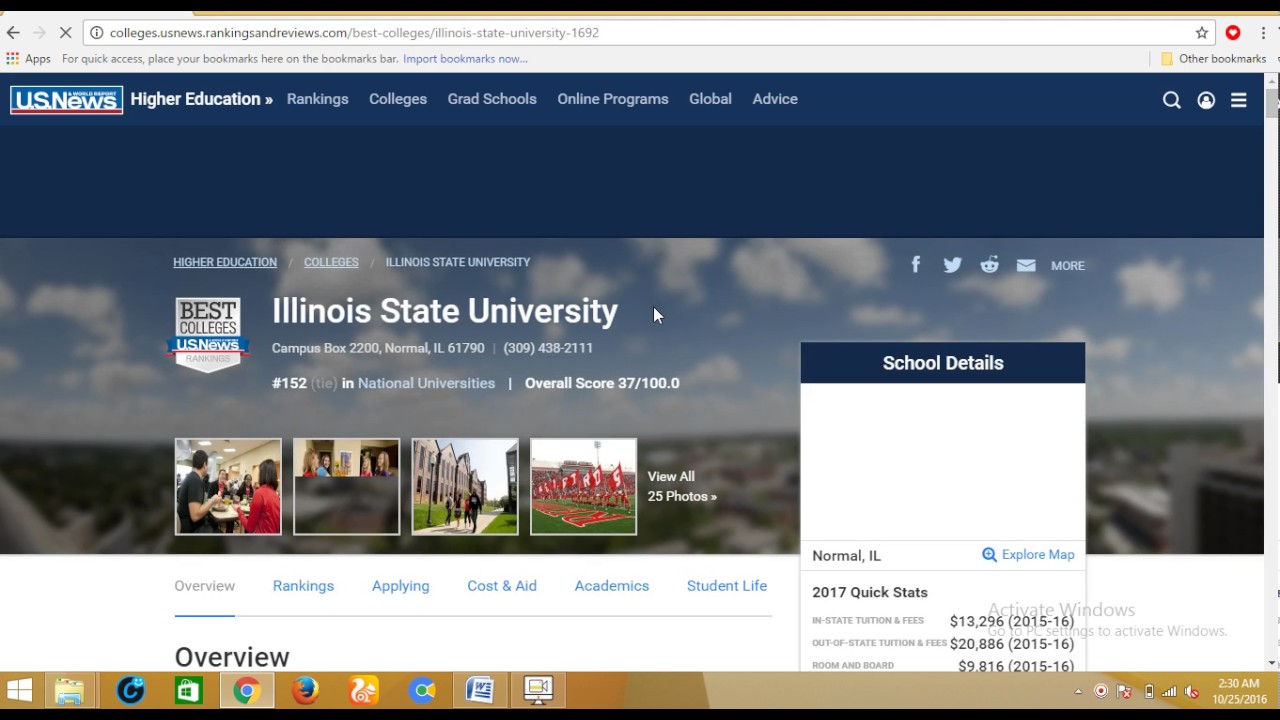The image depicts an open browser window on a Windows operating system, displaying a webpage from US News focused on college rankings. The specific page shown is dedicated to Illinois State University and is part of a series titled "Best Colleges," though it should be noted that this does not necessarily imply high rankings for Illinois State University itself. The university has an overall score of 37 out of 100.

On the left side of the page, there is a badge labeled "Best Colleges," indicating its inclusion in the series. Accompanying the information are several stock photos, showcasing various elements of campus life such as the campus grounds, students in a cafeteria, and other related imagery.

The right side of the page contains sparse school details, including "2017 Quick Stats." Here, the tuition fees are broken down: in-state tuition and fees amount to over $13,000, while out-of-state fees exceed $20,000. Additionally, room and board costs are listed at $9,800. The webpage continues with more details as you scroll down, but the visible portion is cut off.